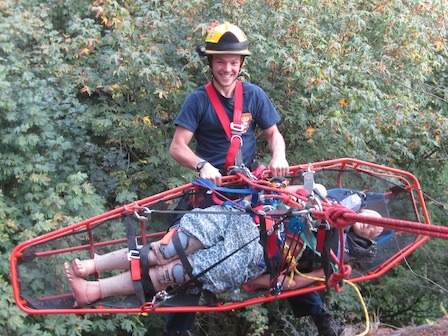In this image, a young man, likely a firefighter in training, is engaged in a practice gurney transport exercise involving rope-based elevation. The young man, who wears a yellow hardhat and a dark blue t-shirt combined with red safety straps, has a broad smile on his face, indicating a sense of accomplishment. He is climbing up a wall with the aid of a rope, keeping a mannequin, dressed in bandages with fake feet, securely positioned on a gurney-like medical evacuation apparatus. The apparatus, resembling a large, oval-shaped, open coffin, is designed to allow safe vertical lifting. In the background, dense brush and leafy trees suggest the setting is in a natural, outdoor environment.